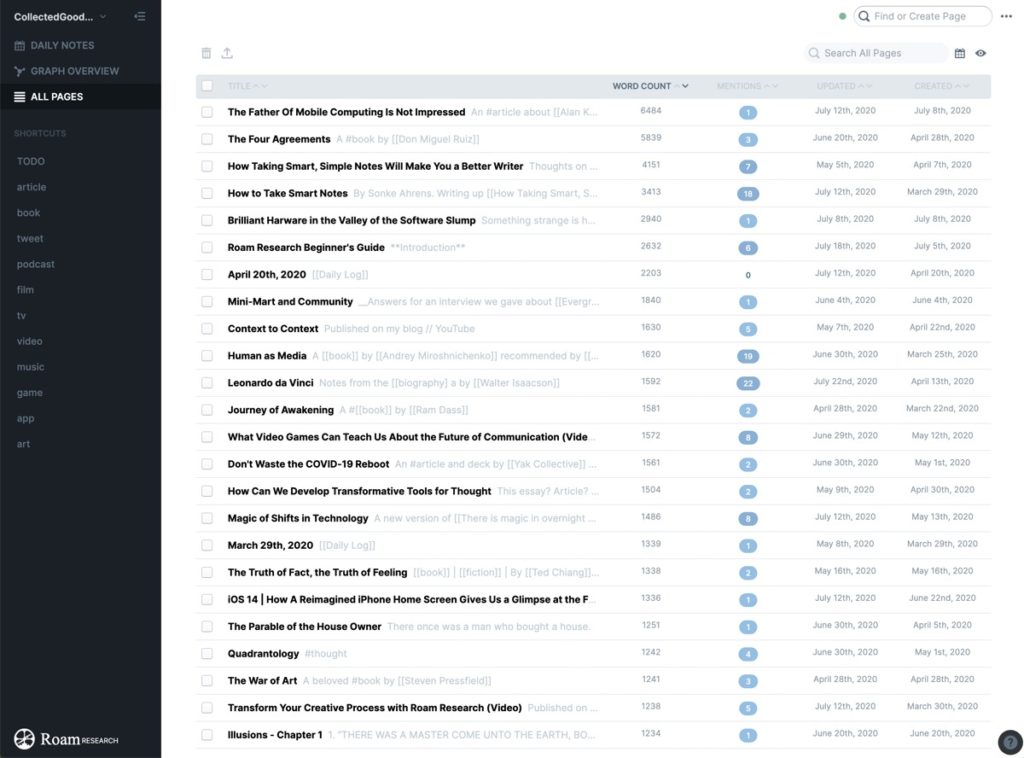The image features a detailed listing of documents related to Rome Research on a white background. On the left side, there is a tall, black, vertical rectangle with white text which includes options such as "Collected Good," "Daily Notes," "Graph Overview," "All Pages," and a "Photo To-Do List." To the right of this black sidebar, there is a vertically arranged list of document titles, each followed by a respective word count, number of mentions, last update, and creation date. 

The documents listed are:

1. "Father of Mobile Computing is Not Impressed"
2. "The Four Agreements"
3. "How Taking Smart Simple Notes Will Make You a Better Writer"
4. "How to Take Smart Notes"
5. "Brilliant Hardware in the Valley of the Software Slump"
6. "Rome Research Beginner's Guide"
7. "April 20, 2020"
8. "Mini Mart in Community"
9. "Context to Context"
10. "Humans as Media"
11. "Leonardo da Vinci"
12. "Journey of Awakening"
13. "What Video Games Can Teach Us About the Future of Communication"
14. "Don't Waste the COVID-19 Reboot"
15. "How Can We Develop Transformative Tools for Thought"
16. "Magic Shifts in Technology"
17. "March 29, 2020"
18. "The Truth of Fact, The Truth of Feeling"
19. "iOS 14"
20. "How a Reimagined iPhone Home Screen Gives Us a Glimpse at the Future"
21. "The Parable of the House Owner"
22. "Quadrantology"
23. "The War of Art"
24. "Transform Your Creative Process with Rome Research"
25. "Video"
26. "Illusions, Chapter 1"

Each title is neatly stacked, providing a clear and organized overview of the contents related to Rome Research.